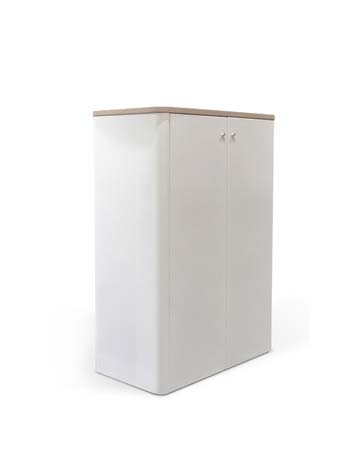In this image, we see a tall and thin white cabinet standing alone against a completely white background. The cabinet, appearing to be around two to three feet tall, features a light brown wooden top, perfect for placing additional items. It is positioned at a diagonal angle, allowing us to see both its side and front. The front of the cabinet showcases two tall double doors that seamlessly fit together, each adorned with a round silver knob near the top. The cabinetry and hardware materials remain undetermined due to a lack of textual description. Shadows cast by overhead lighting are visible around the cabinet, adding depth to the otherwise minimalist setting. This appears to be a standalone kitchen or bathroom cabinet, possibly a stock image meant for home improvement advertising.